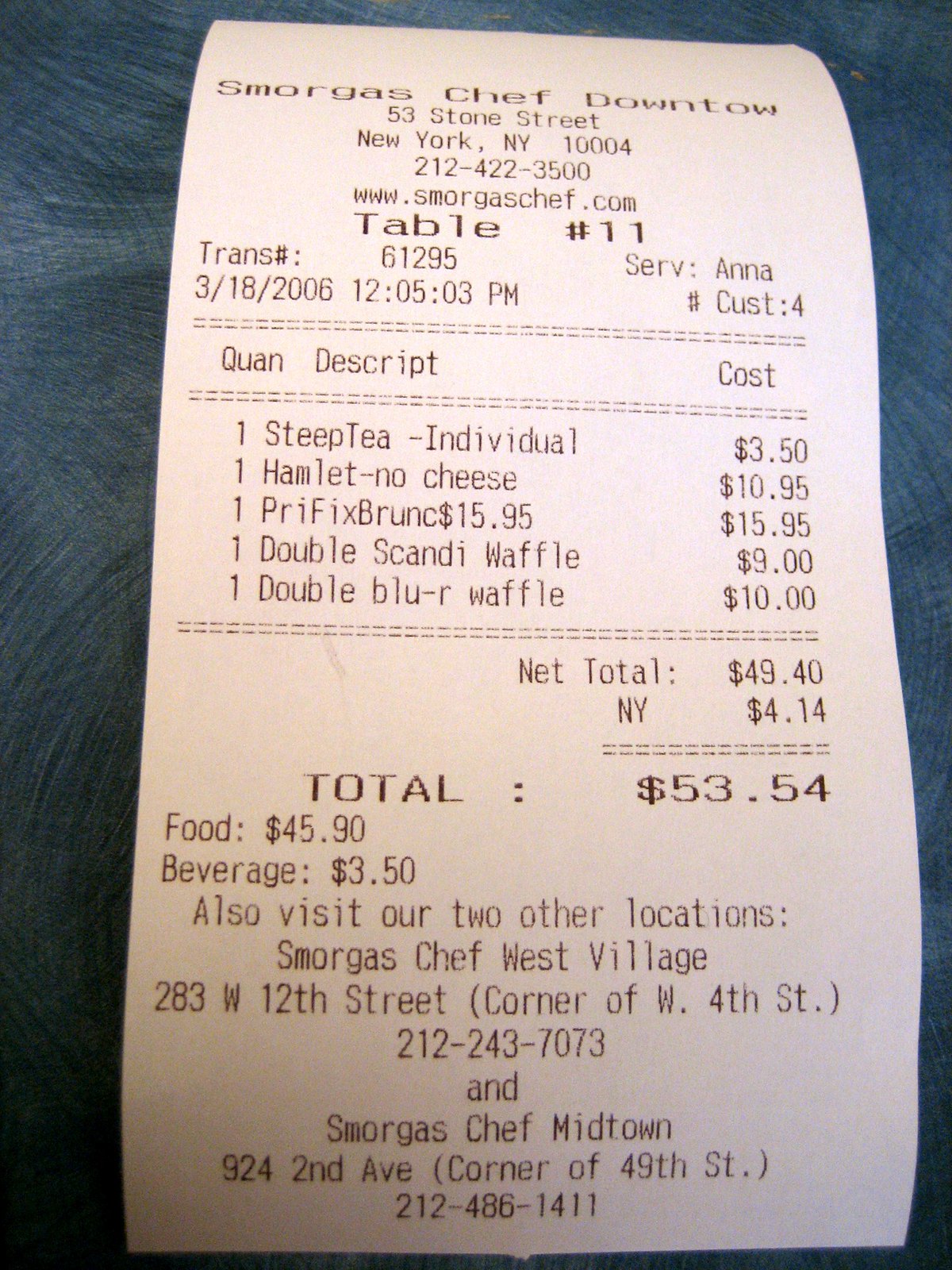A thermal paper restaurant receipt from Smorgas Chef Downtown is prominently featured at the top, with some characters seemingly cut off due to space constraints. The establishment's address is displayed as 53 Stone Street, New York, NY 10004, accompanied by their website, www.smorgaschef.com, and the table number, 11.

The itemized list of ordered dishes includes:
- One Steep Tea (Individual)
- One Hamlet (No Cheese)
- Prefix Brunch
- Double Scandi Waffle (indicating Scandinavian style)
- Double Blue R Waffle (presumably Blueberry)

The subtotal amounts to $49.40, with a final total of $53.54 after tax. Below the total, there's a note suggesting to visit their two other locations, also situated in New York City.